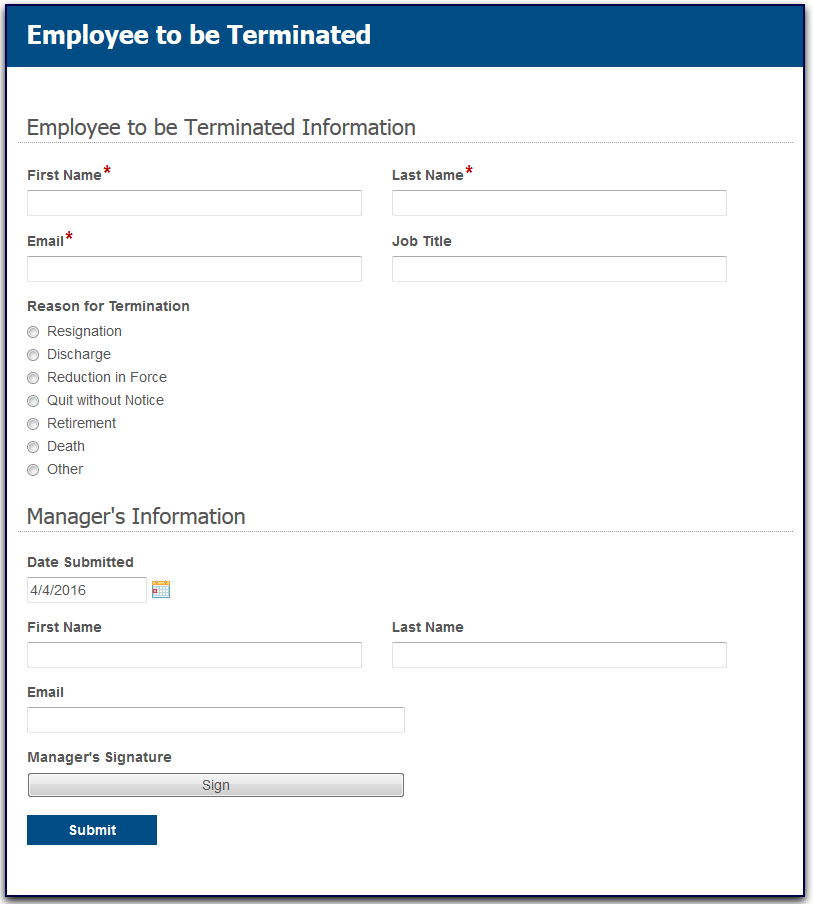The image features a structured form with a dark blue header containing the text "Employee to be Terminated" in white. Below the header, the form is divided into multiple sections on a white background, each outlined by dotted lines.

The first section, labeled "Employee to be Terminated Information," includes fields to input details about the employee. The arrangement is as follows:
- On the left, "First Name" marked with a red asterisk, followed by a text box.
- To the right, "Last Name" also marked with a red asterisk, followed by a text box.
- Below the first name section, "Email" with a red asterisk and a corresponding text box.
- To the right of the email field, "Job Title" with a text box below it.

The next section, titled "Reason for Termination," provides multiple selectable options with checkboxes to the left of each reason. The available reasons are:
- Resignation
- Discharge
- Reduction in Force
- Quit Without Notice
- Retirement
- Death
- Other

Towards the bottom, another section marked by a dotted line and labeled "Manager Information" contains the field:
- "Date Submitted" accompanied by a text box pre-filled with "April 4, 2016" and an adjacent calendar icon.

Overall, the form is designed to systematically gather essential details and categorize the reason for an employee's termination.